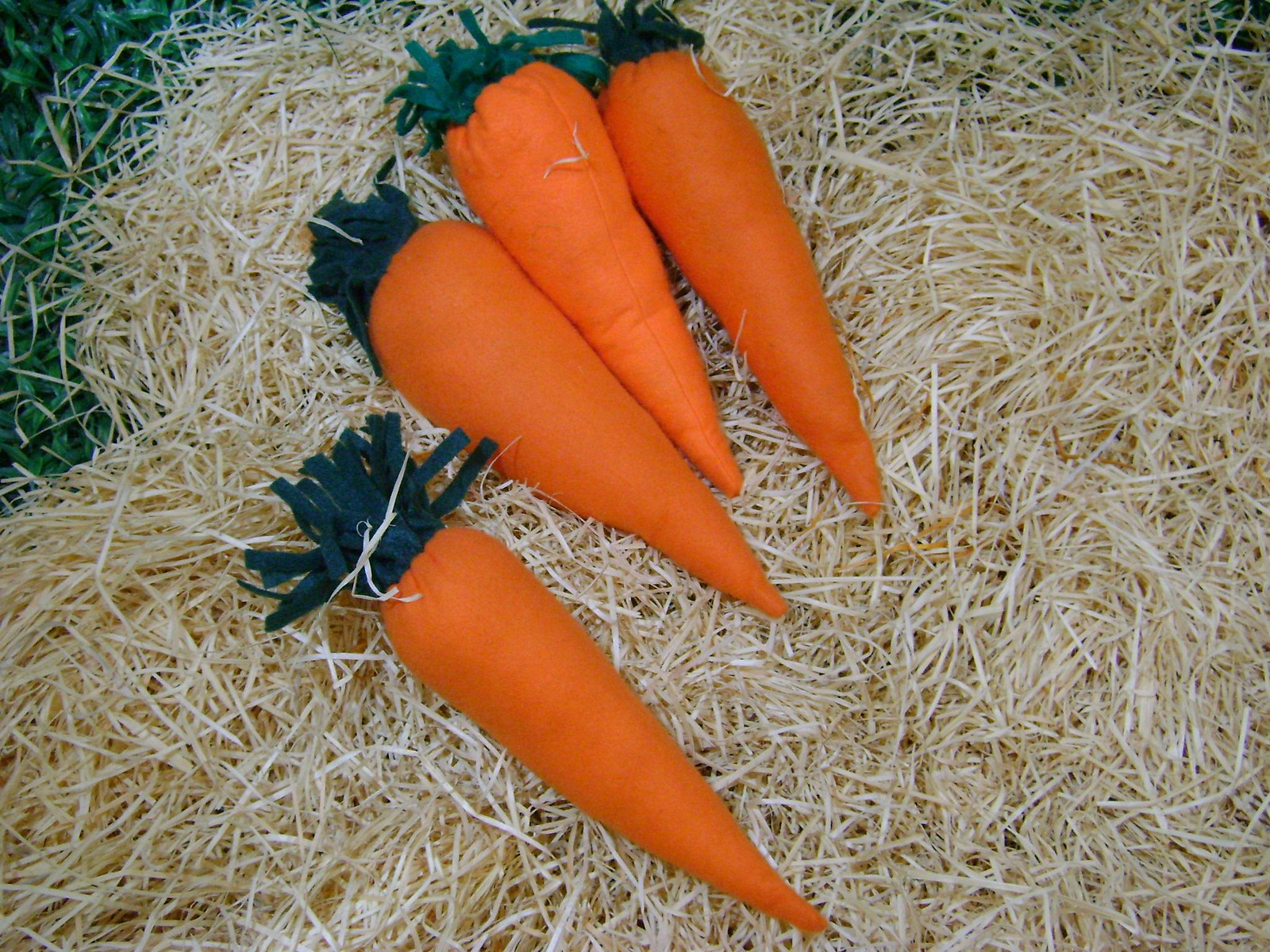This photograph depicts an Easter-themed arrangement viewed from above. The rectangular image, wider than tall, features a soft cream-colored backdrop reminiscent of shredded paper or faux straw, commonly used in Easter baskets. At the corners, especially the top left, patches of traditional green Easter grass peek through, adding a touch of color.

Central to the composition are four whimsical, cloth-stuffed carrots with an orange hue, mimicking the shape and appearance of real carrots — elongated triangles ending in points. Each carrot is adorned with dark green, felt-like material, cut to represent the leafy tops. These fabric carrots are arranged in an inviting, somewhat scattered fashion: three clustered towards the middle top left, with one carrot slightly separated, positioned lower and more to the left.

The detailed stitches and varied orientations of the carrots, with one particularly showing its seam, suggest a handcrafted charm. This playful assortment sits atop the textured, light tan faux straw, creating a delightful and cozy Easter display.